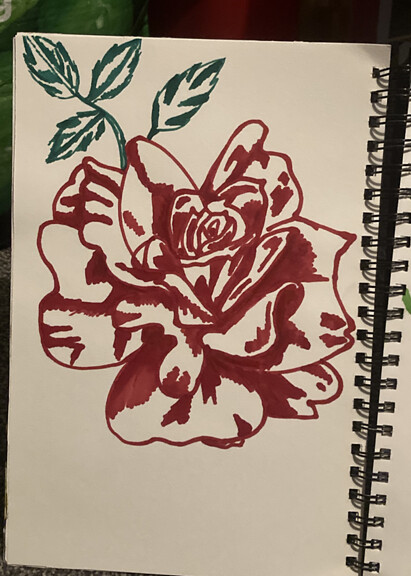This detailed illustration features a close-up view of a rose drawn in a sketchpad with black spiral binding, positioned more towards the upper left corner of the page. The artwork is created using markers, likely permanent ink like Sharpie, which gives it an opaque, slightly matte appearance. The rose itself is intricately outlined and shaded in a deep, maroon-red hue, reminiscent of blood red. The leaves stemming from the rose are carefully lined in green, with some shading that remains uncolored, adding a sense of depth and texture. This sketchbook appears to be made of thicker, mixed media paper to effectively capture the marker's bold pigmentation. The photo is taken in a dimly lit room, which subtly mutes the vibrancy of the red and green colors, adding an intimate and moody ambiance to the image.